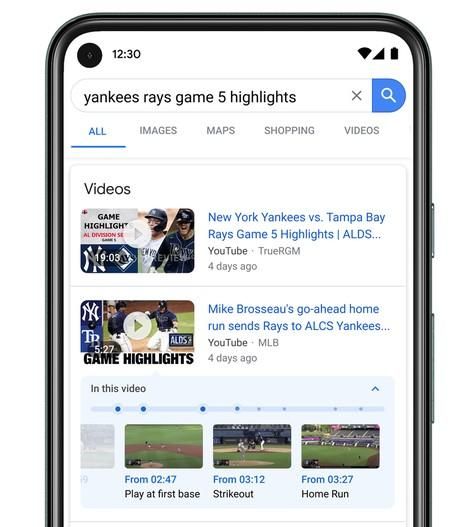The image depicts the bottom half of a cell phone with the very bottom edge cut off. The device is shown with a physical case, clearly visible on the left-hand side of the phone. On the right side of the image, which corresponds to the left side of the cell phone, there are physical buttons. The cell phone is displaying a Google search page, with the search query "Yankee Rays game five highlights" visible in the search bar. Below the search bar, a horizontal menu shows various options: All, Images, Maps, Shopping, and Videos, with the "All" tab currently selected.

Underneath the horizontal menu, there are two notable search results labeled "Videos." The first video on the upper left is titled "New York Yankees vs. Tampa Bay Rays Game Five Highlights," posted four days ago by the YouTube user "True RGM." The second video is titled "Mike Brosseau's go-ahead home run sends Rays to ALCS Yankees," also from YouTube, and posted by the MLB.